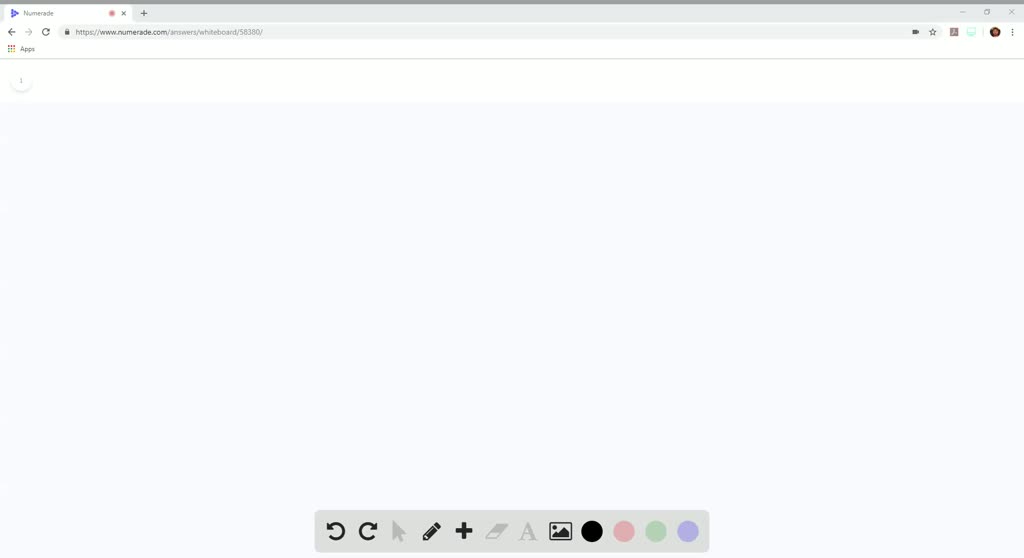The image displays a web browser interface, specifically Google Chrome, with a whiteboard application open in full screen. The background of the whiteboard is a light gray color, providing a neutral backdrop for the content. Along the bottom of the screen, a toolbar contains multiple icons, including a mouse pointer, a pencil, a plus sign, an "A" representing text, and an image icon, among others. These icons indicate various tools and functionalities available for use within the whiteboard application, organized into distinct sections for easy access.